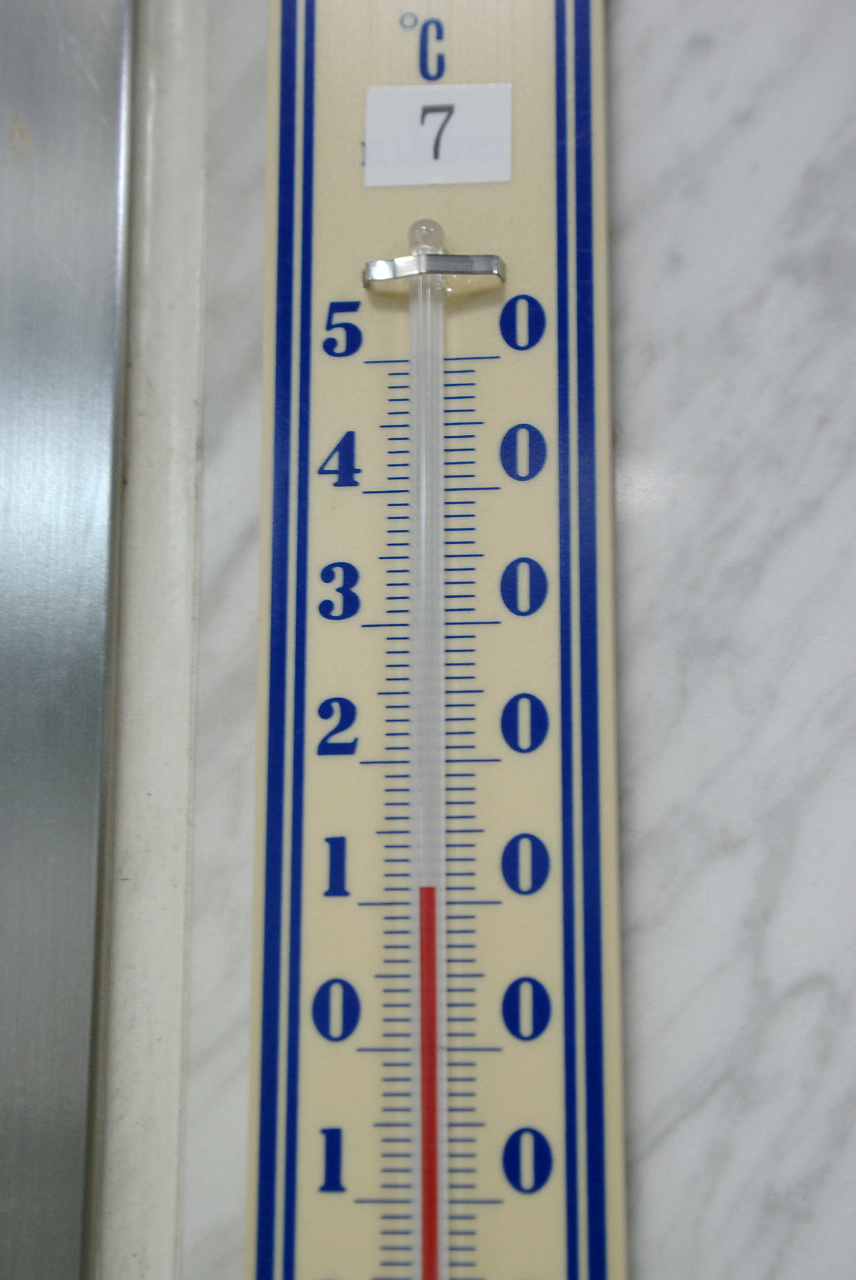This image features a detailed view of a thermometer positioned vertically against a surface that appears to be a granite wall. The thermometer displays blue numerical markings, with the scale marked in degrees Celsius. At the top of the thermometer, the letter "C" is prominently visible, indicating the Celsius scale. Below this, the scale starts at a double zero (00) and increments by tens with numbers 10, 20, 30, 40, and 50, all in blue. Between these larger increments are smaller blue markings representing single units.

A distinct red line within the thermometer indicates the temperature, which is currently reading 11 degrees Celsius. Additionally, there is a white label situated just below the "C" and above the lower end of the thermometer, featuring a black number 7. This label provides additional information, possibly related to the thermometer's calibration or model number. The overall image captures the precision and detailed markings of the thermometer against the textured backdrop.